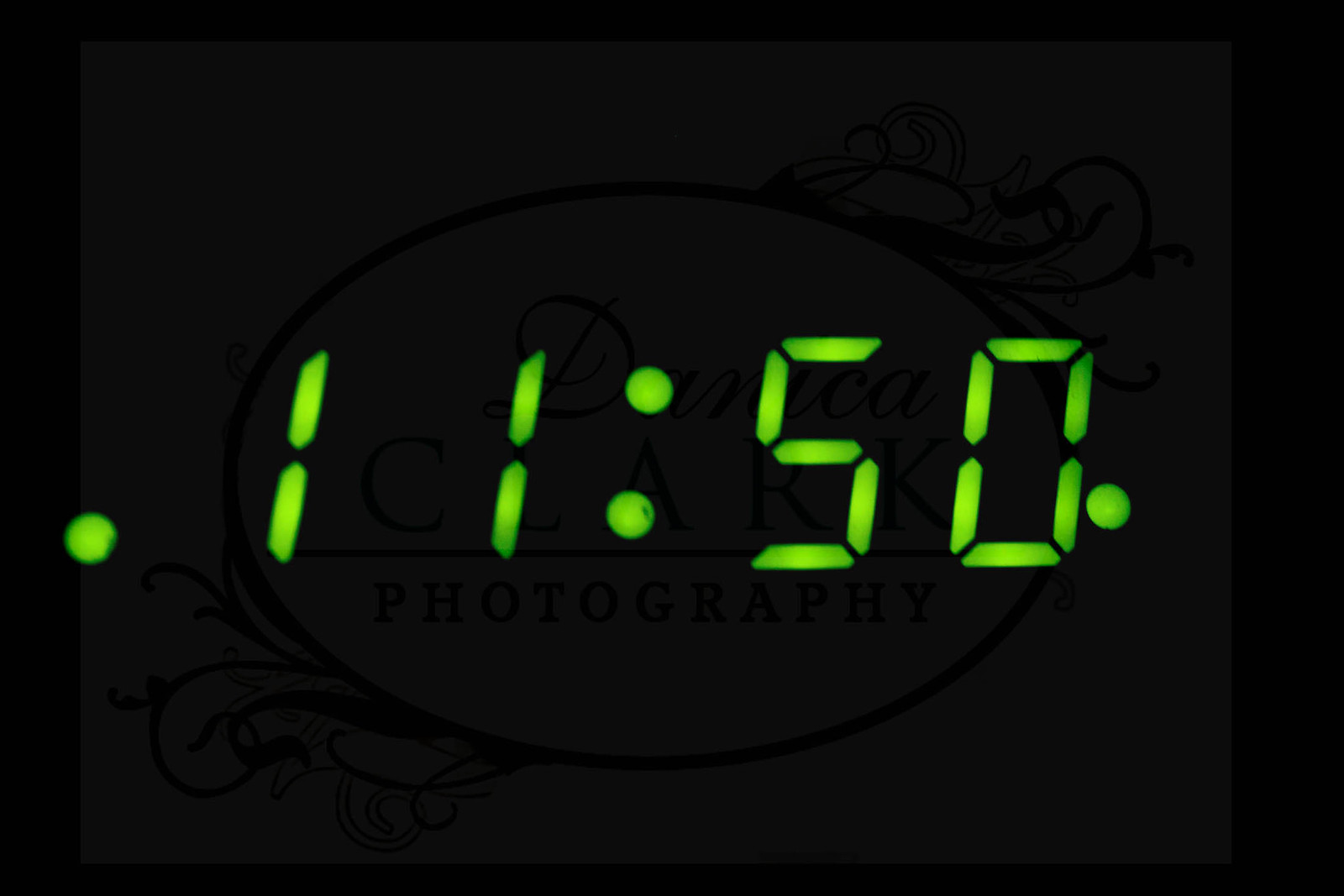On a deep black background, there is a subtle, oval-shaped watermark at the center, etched with delicate ornamental details. The watermark features the word "Photography" prominently inscribed in the middle. Extending from the top and bottom of the oval, intricate designs resembling small leaves and flowers add an elegant touch. Surrounding this central feature, a green dot is placed followed by the number "1150" and another green dot, symmetrically arranged. Additionally, delicate swirls akin to branches and leaves embellish the design on both the top and bottom, enhancing the overall aesthetic.